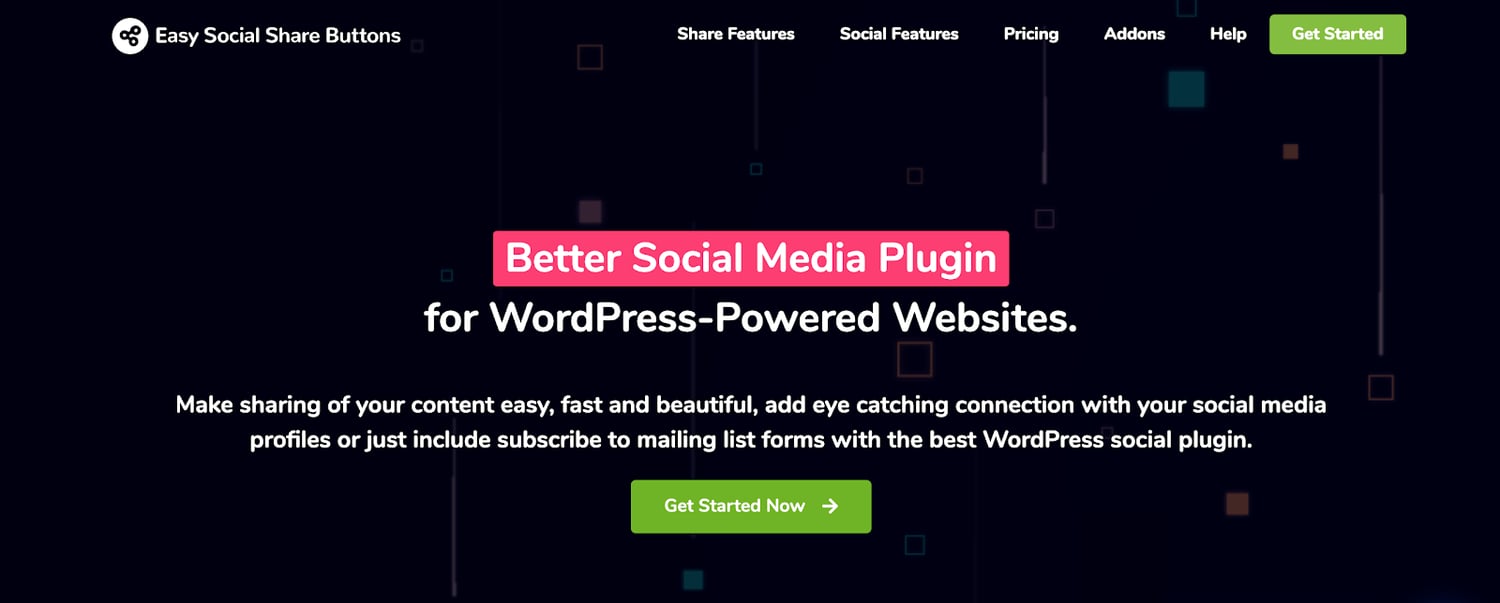The image features a predominantly black background. Positioned in the upper left corner, a circular icon with three smaller black circles connected by lines is displayed, accompanied by the text "Easy Social Share Buttons." 

To the right, a series of options is listed: "Share Features," "Social Features," "Pricing," "Add-Ons," "Help," and "Get Started." The "Get Started" option is highlighted within a green rectangle with white text.

Dominating the center of the image is a dark pink banner, prominently displaying in white text, "Better Social Media Plugin." Below this banner, against the black background, additional white text reads, "For WordPress-powered websites," with "WordPress" correctly shown in one word with capitalized 'W' and 'P.'

Further down, the description continues: "Make sharing of your content easy, fast, and beautiful. Add eye-catching connection with your social media profiles or include subscription forms with the best WordPress social plugin." 

At the bottom, a green button with white text, "Get Started Now," is featured, along with an arrow pointing to the right.